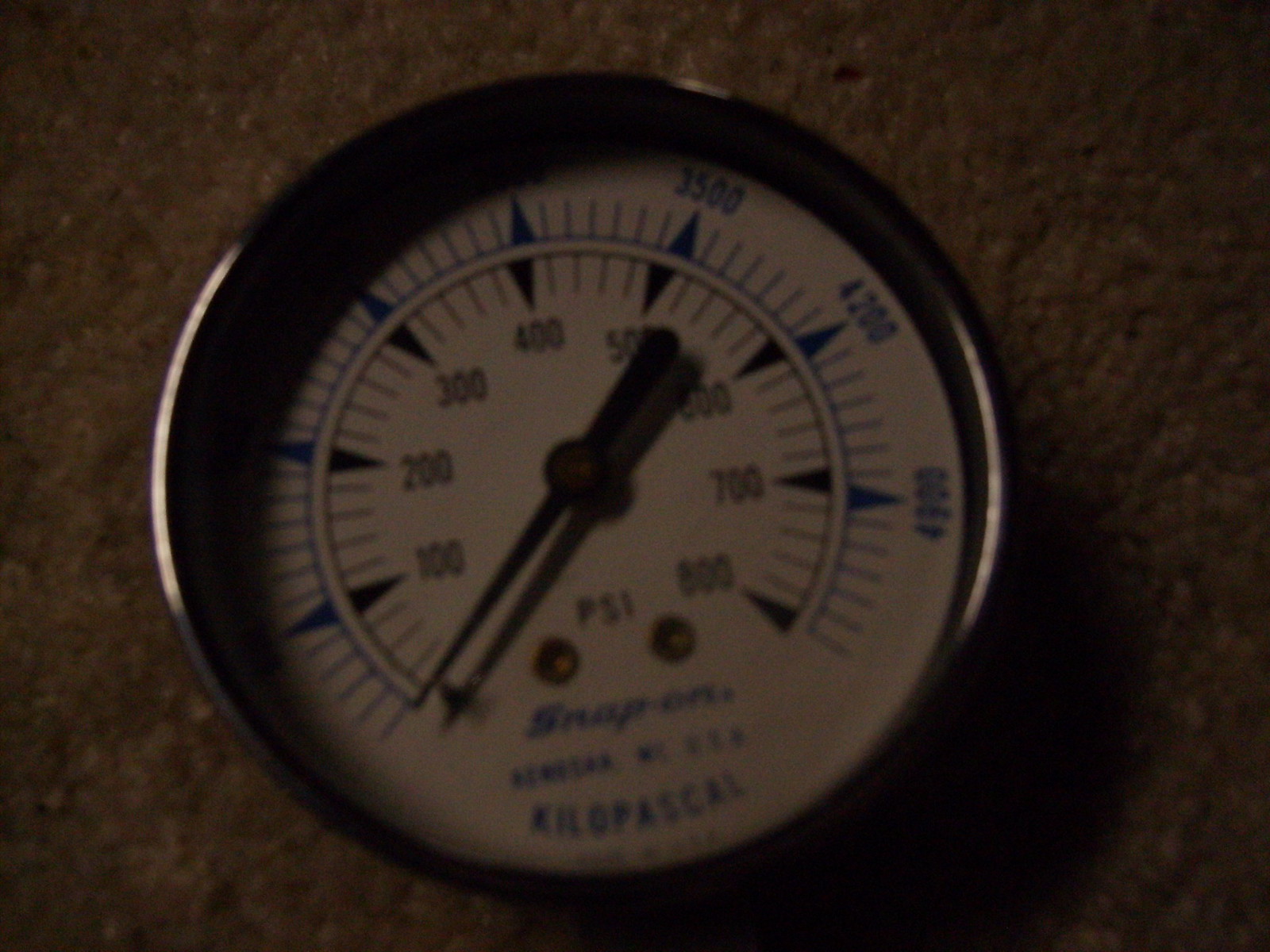This image captures a blurry and dimly lit photo of a pressure gauge. The gauge is circular with a silver metal rim and is positioned on what appears to be a rough, brown surface that could be rock or concrete. Due to the poor lighting, the background texture is hard to ascertain. 

The gauge's face has a white background with a blue circular dial that occupies most of the interior. Around 80% of the circumference of the dial is marked by a double line, which is open at the bottom. Blue hatch marks encircle the dial, with every sixth hatch mark featuring a blue diamond shape behind the lines. A blue triangle indicates different measurements along the dial.

The needle on the gauge is currently pointing to zero. There are two concentric levels of measurements within the circle. The inner scale reads 100, 200, 300, 400, 500, 600, 700, and 800, progressing from left to right around the dial. On the outer part of the dial, the numbers start at 3,500 at the top right and continue with 4,200 and 4,900 visible as they arc around the gauge. The left side of the dial is obscured by shadows, making those numbers indiscernible.

Below the needle, the gauge is labeled "PSI," and further down in blue letters, it reads "Snap-on." The additional text appears to reference "Kenosha, Washington" or possibly "Kilo Pascal," although the low image quality makes this uncertain.